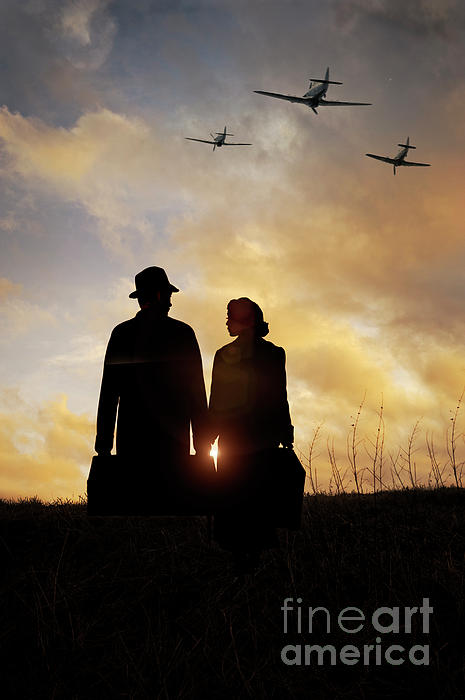This evocative piece from Fine Art America presents a picturesque yet haunting scene. Dominating the top two-thirds of the canvas is a mesmerizing sunset, painted with hues of yellow, gray, and blue, interspersed with dramatic clouds. The lower third of the image is a dark brown grassy field, indicating a sense of ground beneath a vast, open sky. In this setting, three World War II-era fighter planes fly in a precise triangular formation above, adding a historical and perhaps ominous touch to the artwork.

Central to the piece, where the field meets the sky, stand a man and a woman, their dark silhouettes stark against the setting sun. The light deftly streams between their clasped hands, illuminating their forms. The man, noticeably without legs as though incomplete, holds an additional briefcase and wears a hat and trench coat, while the woman in her trench coat remains fully visible. Both figures are well-dressed, each carrying a suitcase, encapsulating a narrative of escape or journey.

The overall composition, with its surreal touches such as the missing legs and the crisp historical planes, gives an impression of an AI-generated image or a stylized movie poster, reinforcing a story of departure and uncertainty, perhaps hinting at a wartime escape. The Fine Art America watermark in the bottom right corner subtly authenticates the source of the artwork.